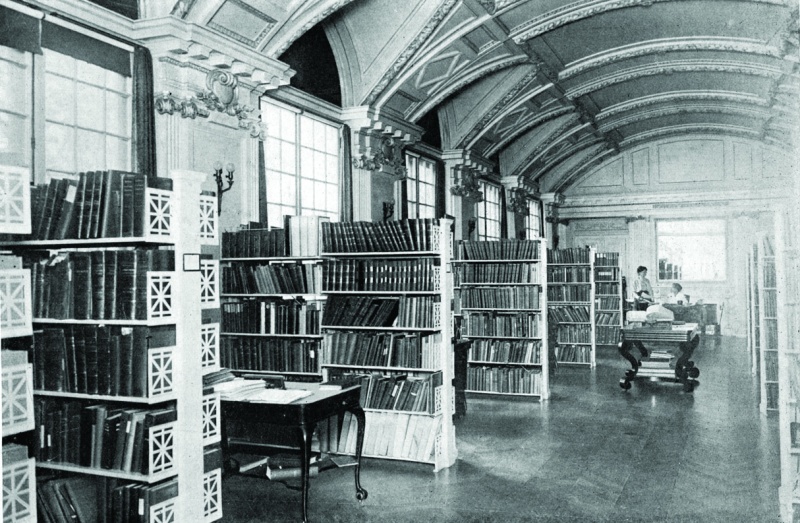This black and white vintage photograph captures the interior of an ornate library with an arched ceiling approximately 15 to 20 feet high. The library is adorned with intricate wood carvings around the arches and large windows that stretch nearly from the floor to the ceiling on the left side of the room. Bookshelves packed with books line both the left and right walls, with support columns situated between the windows on the left side, each column accompanied by a bookshelf. In the central walkway, we find a distinctive wooden table with zigzag-shaped legs, and a shiny tiled floor reflecting the classic ambiance of the space. Toward the back of the library, two women are engaged in conversation; one is seated at the library desk, and the other stands nearby. There are also additional desks and tables distributed throughout, enhancing the historic and scholarly atmosphere depicted in this rectangular image.